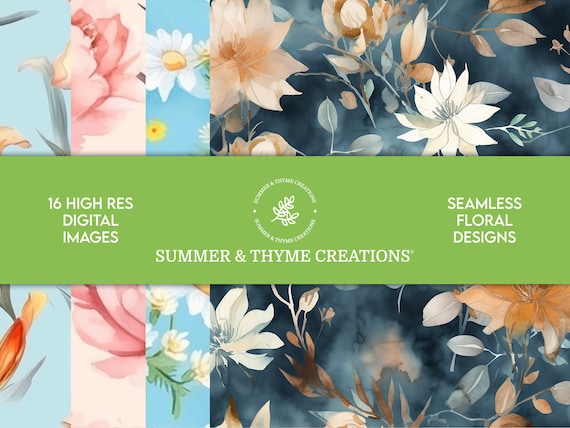The advertisement image showcases "16 High-Res Digital Images" with a prominent green band running horizontally across the center. In white text within the band, it reads, from left to right: "16 High-Res Digital Images," "Summer and Thyme Creations," and "Seamless Floral Designs." Centrally placed in the green band is a circular logo featuring a white stamp of the herb thyme, encircled by the phrase "Summer and Thyme Creations" repeated twice with dots in between. The background is divided into four distinct sections featuring an array of floral designs. The largest section, positioned slightly off-center, has a grayish-blue background adorned with pink and white flowers. To its left is a vertical pink band featuring pink flowers. Further left is a vertical light blue band with white daisies. On the far left is a vertical light blue section with orange flowers against a grayish background. The floral patterns and colors create a vibrant, seamless design that beautifully complements the detailed product description in the central green band.